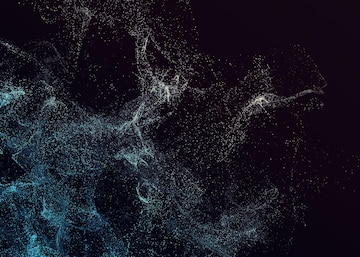The image presents an abstract piece of art on a solid black background, featuring intricate patterns that transition between blue and white hues. On the left side, blue specks and clusters dominate, resembling sand or fine droplets suspended in mid-air. This blue gradually fades into white as it approaches the center and right side of the image, with the white concentrations reaching almost to the top and close to the right edge. The blue regions primarily occupy the bottom left, rising up about three-quarters of the way. The individual dots or specks give the appearance of either smoke, water droplets, or sound waves, contributing to a highly abstract and visually engaging composition. The image has a minimalist yet detailed aesthetic, capturing a snapshot that suggests fluidity and movement within a static frame.